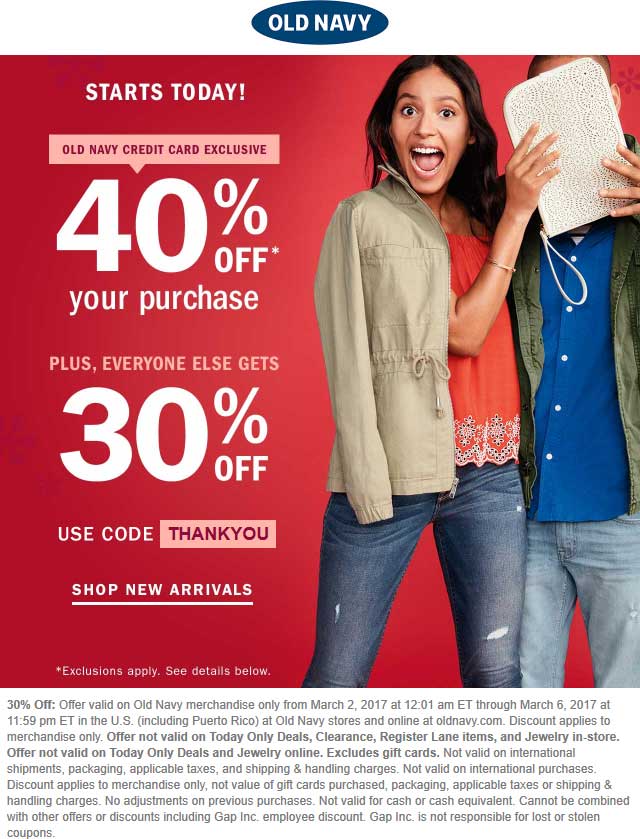An elderly woman and a man pose excitedly in a promotional image for Old Navy. The woman, with a wide, joyful smile, has a jacket draped over her shoulders, pairing it with blue jeans. She holds a shopping bag that partially obscures the man's face. The man, dressed in a blue button-down shirt and a green bomber jacket, also wears blue jeans. To the left, a blue oval contains the text: "Starts Today, Old Navy Credit Card Exclusive 40% Off Your Purchase, Plus Everyone Else Gets 30% Off. Use Code THANKYOU. Shop New Arrivals."

Below this, in smaller text, it reads: "Exclusions apply. See details below." The bottom section contains tags outlining the offer specifics: "30% off offer valid on Old Navy merchandise only from March 2nd, 2017 at 12 am ET through March 6th, 2017 at 11:59 pm ET in the US, including Puerto Rico, at Old Navy stores and online at oldnavy.com. The discount applies to merchandise only, excluding 'Today Only' deals, clearance, register lane items, jewelry, and gift cards." Additional exclusions and terms continue in the fine print.